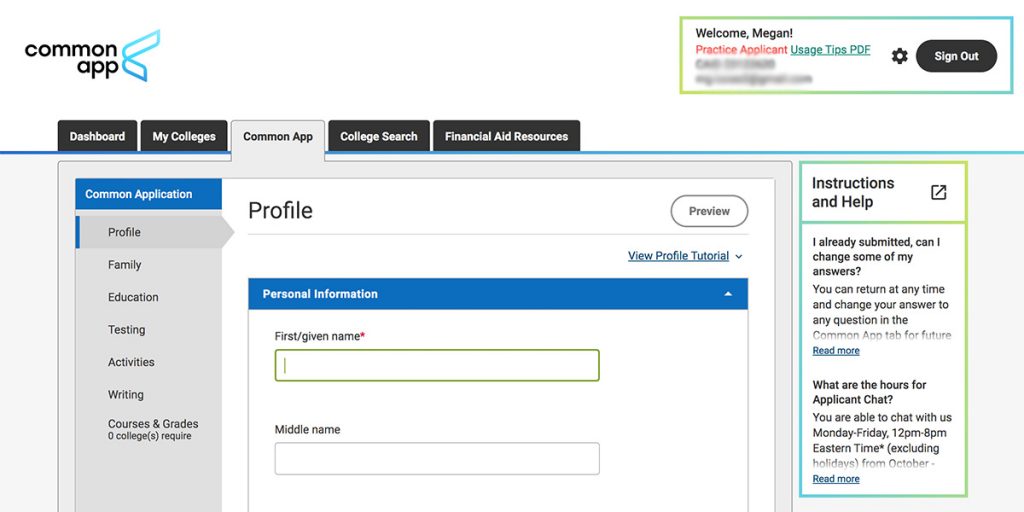A partial screenshot of the Common App website is depicted, showing truncated sections of the interface. The header clearly displays "Common App" with "Common" on top and "App" below. Accompanying the text is an icon, presumably the organization's logo.

On the right side of the screen, there is a two-toned boxed area with colors aqua green and a hint of orange. This section greets the user with "Welcome Megan" on the left, followed by "Practice Applicant" in red font, and a link labeled "Usage Tips PDF." To the right, an oval button reads "Sign Out."

The left-hand navigation pane lists several tabs: Dashboard, My Colleges, Common App, College Search, Financial Aid Resources, with the Common App tab being open. Underneath the heading "Common Application," which is highlighted in blue, there are subcategories such as Profile, Family, Education, Testing, Activities, Writing, Courses and Grades.

In the main content area, it mentions "Zero Colleges (S Require)" and showcases the "Profile" section centrally positioned. Adjacent to the "Profile" tab on the right is an oval "Preview" button. The "Personal Information" section below has fields for the first name and middle name. To the right of these fields, there is a section labeled "Instructions and Help."